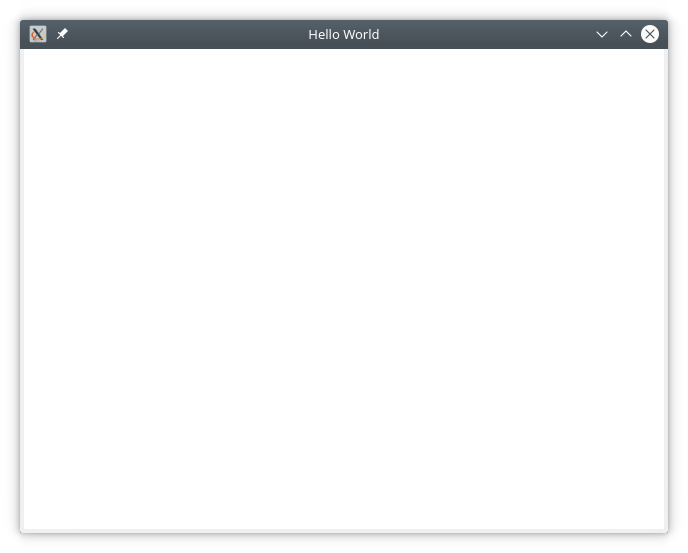A screenshot displays a predominantly white screen with a potential error, as almost the entire screen is blank. The only visible elements are at the top, where a dark gray header bar spans across. Within this header, there is a gray square containing a dark gray "X" and a white pushpin icon. Situated centrally within the header is the text "Hello World." To the left, there are up and down arrows, and a dark gray "X" icon encased in a white circle. The top of the screen is outlined with a gray border, further distinguishing the header from the rest of the blank white screen.